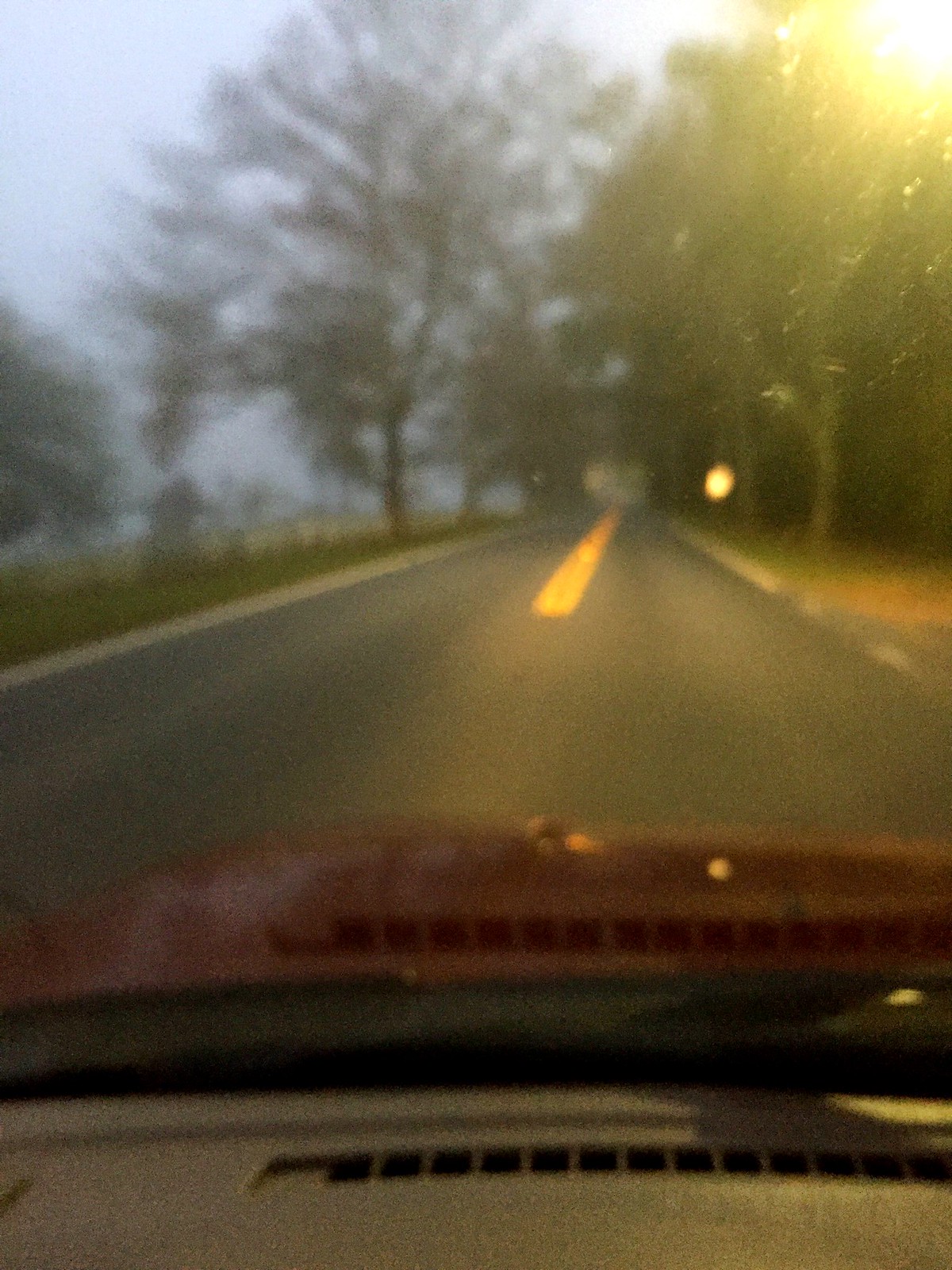This portrait-style image, taken in a vertically aligned profile, captures a blurry and grainy scene from inside a car, looking out through the windshield. The photograph depicts a nightfall or early evening setting on a two-lane road, where the car is driving on the right side, closely approaching a long yellow line that divides the lanes. The front hood of the car is discernibly red. 

Off to the left side of the road, leafless trees can be seen, while on the right side, the trees still have leaves. The ground surface appears as gray cement, adding to the scene's overcast ambiance. There's a bright yellow streetlight shining through from the top right corner of the image, illuminating parts of the scene and casting light onto the windshield. The top of the car's dashboard is faintly visible at the bottom of the image, adding to the internal perspective of the photograph.